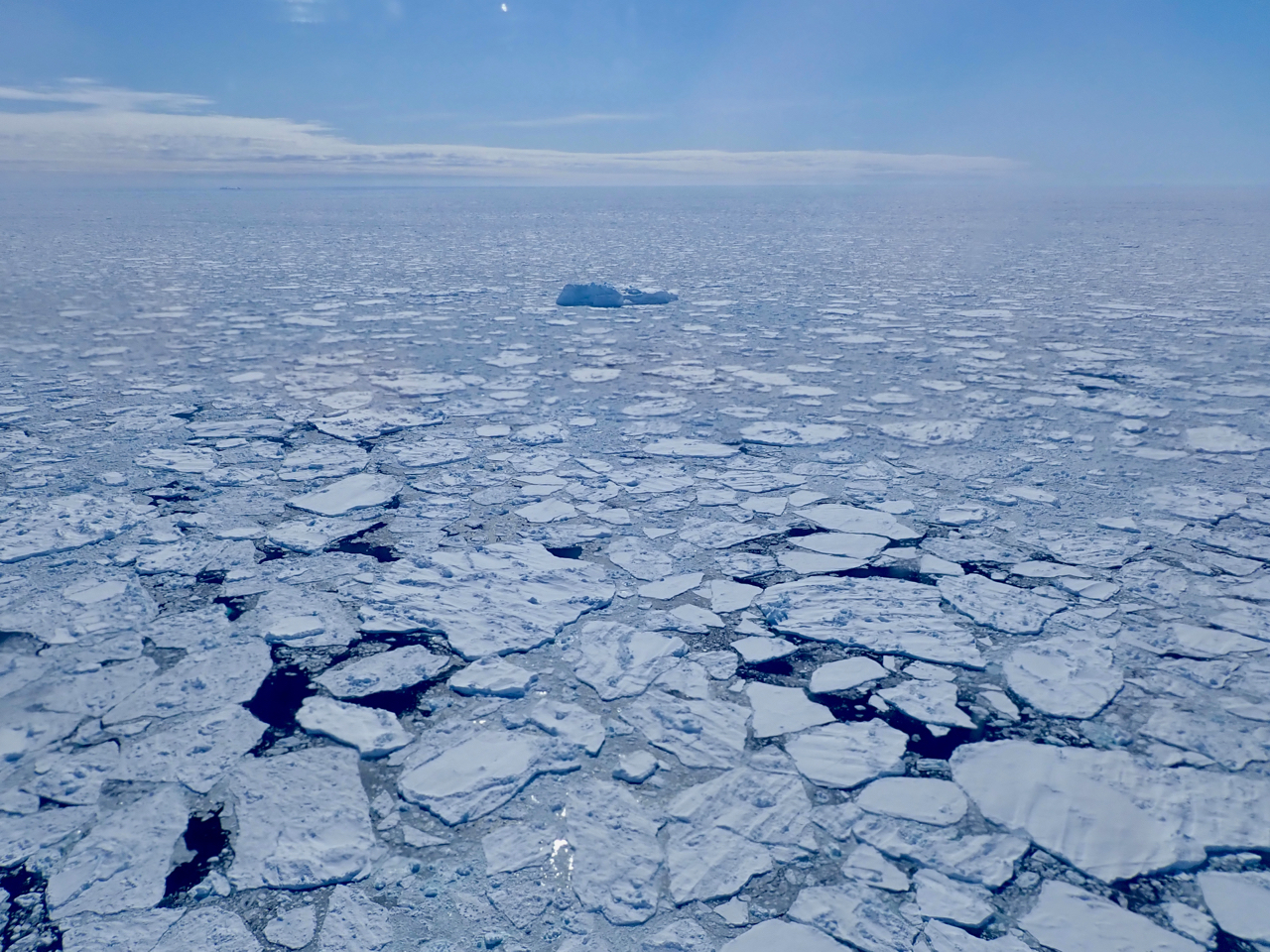The image depicts a vast, desolate landscape dominated by various shades of blue and grey. The ground is notably craggly and fractured, featuring flat tablets of stone or possibly clay scattered throughout. The terrain appears to be reminiscent of either a cold, icy desert or a hot, arid one, with broken and cracked surfaces extending far into the horizon until they blend seamlessly with the skyline. In the backdrop, a subtle gradient of pink and blue suggests that the sun may have just set, casting a soft light across the scene. Amidst the cracked ground, there is a lone, ambiguous object towards the middle—potentially a rock, a tent, an iceberg, or even a dead tree—standing as a solitary figure in this otherwise barren expanse. The sky above is graced with a few passing clouds, adding to the overall impression of a frozen or heat-scorched wasteland, empty and silent.